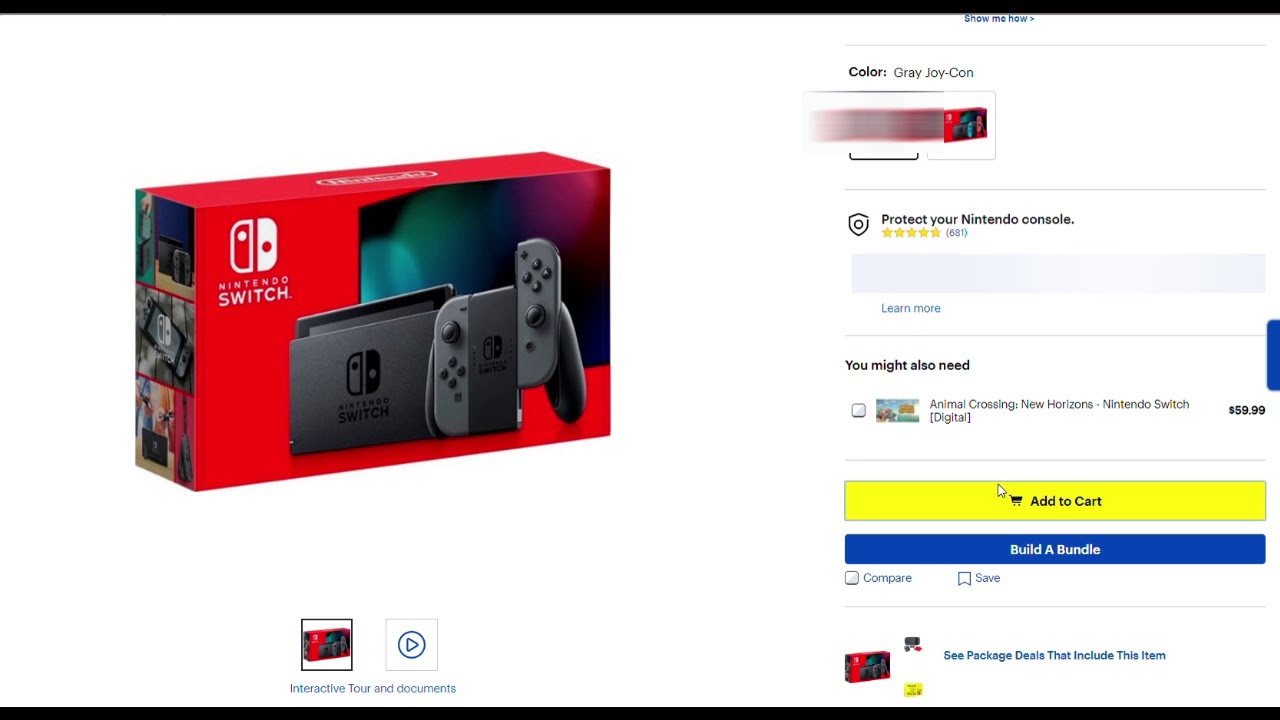The image appears to be a webpage with a clean, white background. Thin black lines span the width of the page at both the top and bottom, leaving the sides unbounded. Dominating the upper half of the page is an image of a red Nintendo Switch box. A black Nintendo Switch console is depicted on the box, along with matching black Joy-Con controllers. The box also portrays a TV in the corner, suggesting connectivity. Additionally, there's a handheld controller grip for the Joy-Cons.

To the right of the Switch box, small gray text reads "Joy-Con." Below this text is a slightly blurred image of the Nintendo Switch box, followed by an icon of a shield with the text "Protect Your Nintendo Console" underneath. Further down, the phrase "You Might Also Need" introduces an image of the game "Animal Crossing: New Horizons," priced at $59.99. Below the game description, a bright yellow rectangular button reads "Add to Cart." Beneath this, a blue button labeled "Build a Bundle" is visible.